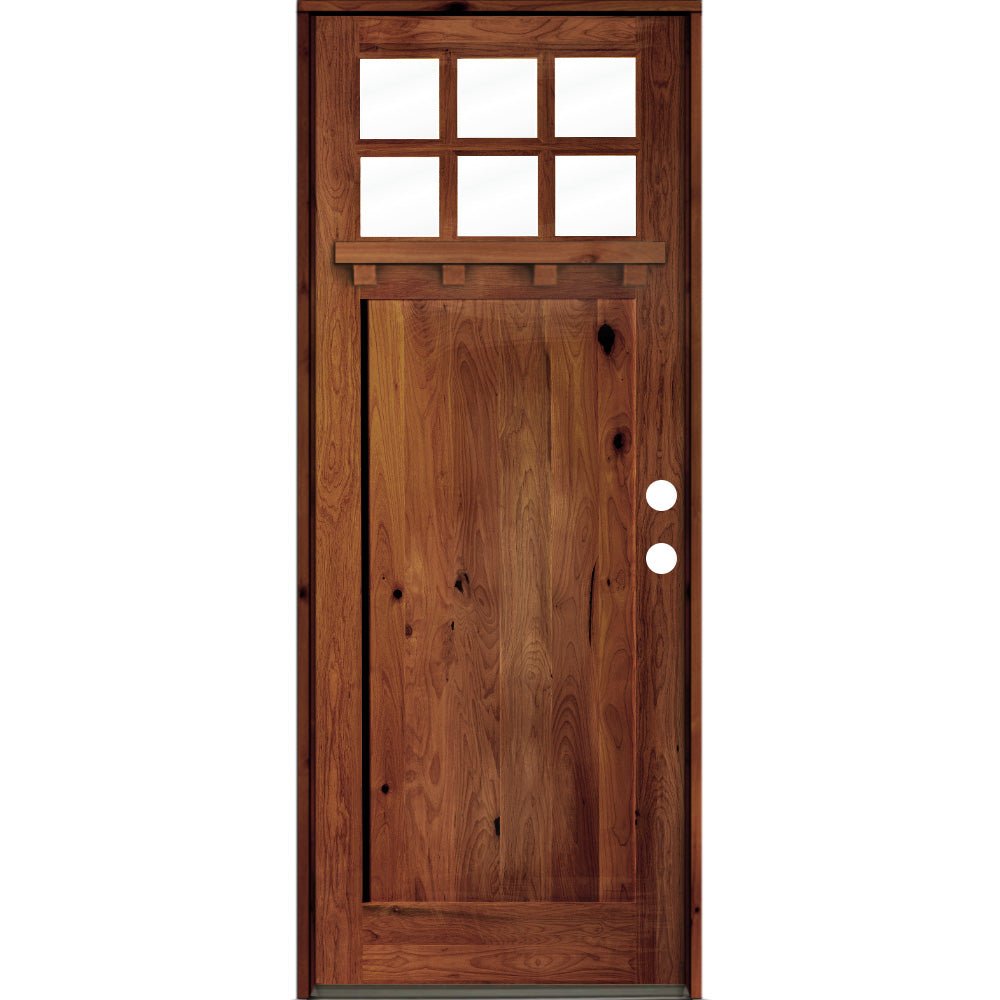This is a detailed image of a long, rectangular, medium-varnished wooden door, positioned vertically. It prominently features six clear glass window panes at the top, arranged in two rows of three squares. Below these windows, there are additional wooden panels that add to its intricate design. Two holes are cut into the right side of the door for a deadbolt lock and a doorknob, although the hardware is currently missing. The wood grain is clearly visible, enhancing its detailed appearance, and a small stripe of green can be seen at the bottom. The door's dark wood hue and the framed structure add to its detailed and somewhat digital look, emphasizing its architectural craftsmanship.